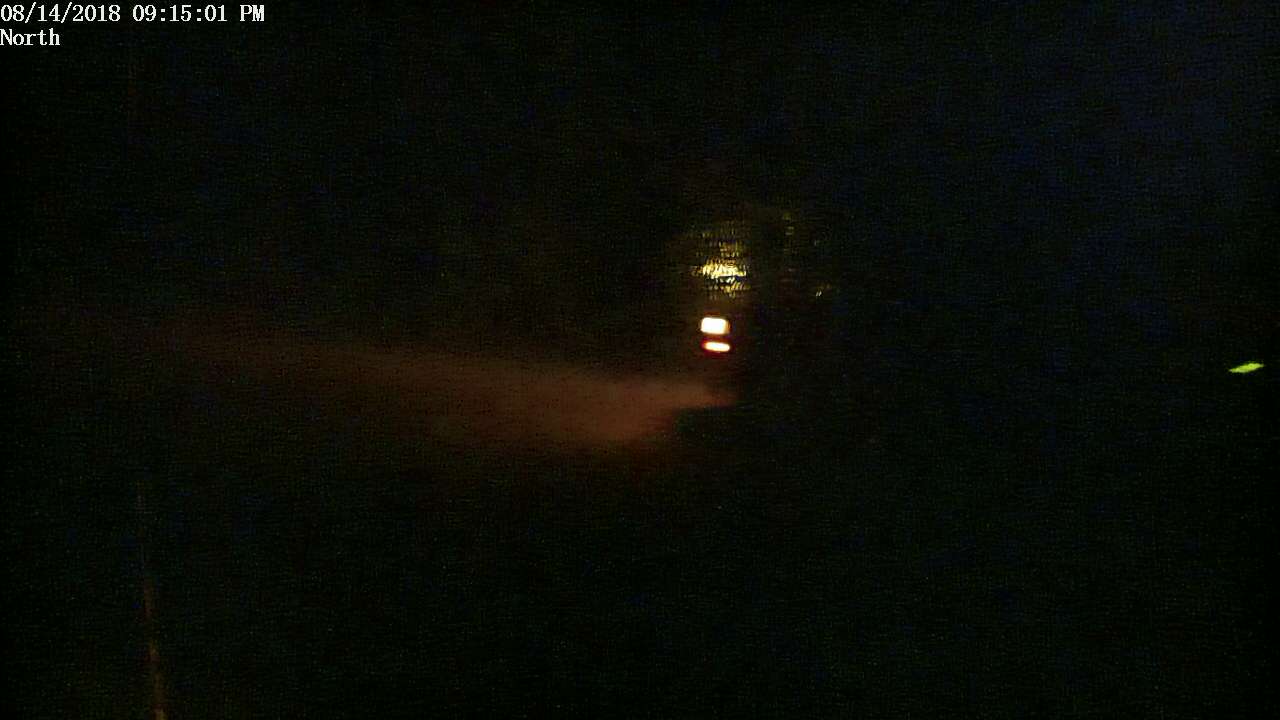In this nighttime image, taken outdoors on August 14, 2018, at 09:15:01 PM, a timestamp and the word "north" are visible in the upper left-hand corner. The photograph is quite dark and slightly grainy, revealing little detail. However, at the center, there appears to be a pair of rectangular lights, suggestive of vehicle headlights or possibly the taillights of a motorcycle. These lights cast a faint illumination on the ground, which might be grass or a road, showing a narrow stretch of light heading leftward. To the right side of the image, a small, glowing rectangle can be seen. Above the two main lights, there is a barely discernible object that could be interpreted as the back of a person's coat. Despite the clarity issues, these light sources are the defining features in an otherwise obscure scene.